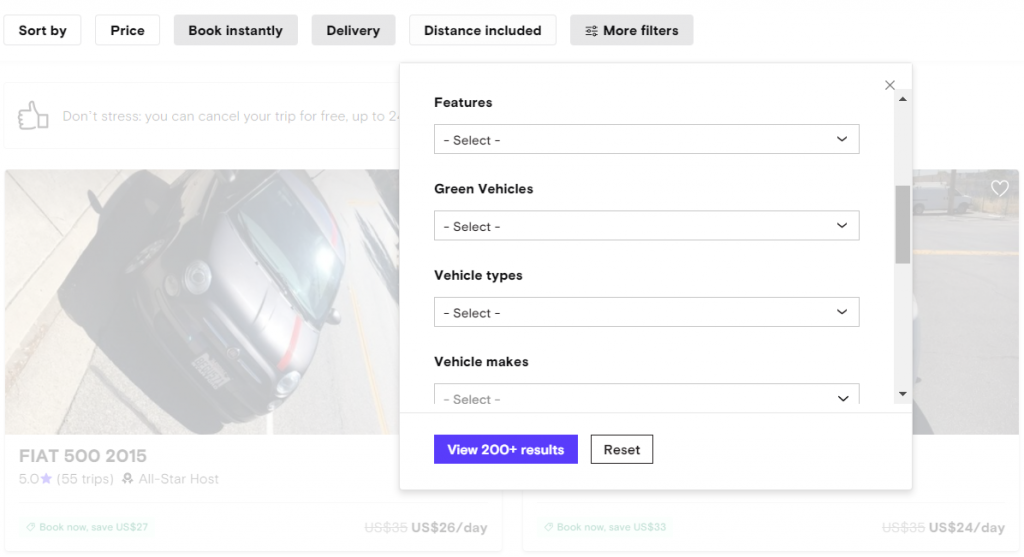This detailed screenshot captures the interface of a car rental app showcasing a hazy, angled photograph of a Fiat 500 from 2015. The photograph suffers from poor clarity and excessive reflection. Directly beneath the image, the details reveal a high rating of 5.0 stars accumulated over 55 trips and an "All-Star Host" designation. An adjacent thumbs-up icon reassures users with the message: "Don't stress, you can cancel your trip for free." 

Above the image, several interactive buttons provide users with various rental options: "Sort by," "Price," "Book Instantly," "Delivery," "Distance Included," and "More Filters." Further down, a section labeled "Features" includes a dropdown arrow, inviting users to explore the vehicle’s specifications. This is followed by additional customized dropdown menus for "Green Vehicles," "Vehicle Types," and "Vehicle Makes."

At the lower part of the screenshot, two prominent blue buttons allow users to either "View 200+ Results" or "Reset" their selections, facilitating a comprehensive and user-friendly car booking experience.